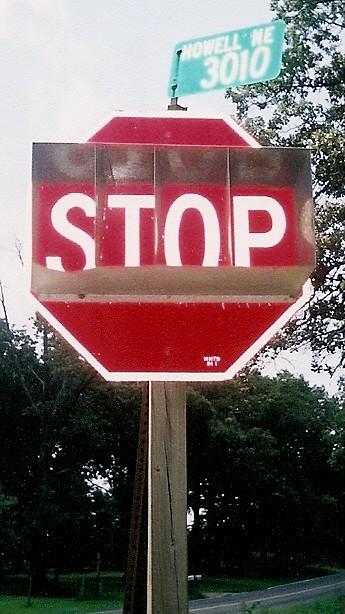This photograph captures a unique street corner scene featuring a weathered, dark gray-brown wooden post supporting a vintage stop sign. Unlike typical metallic poles, this sturdy post gives a rustic feel to the setting. The stop sign itself is traditional in shape and color, sporting the usual red background with bold white letters spelling "STOP," but it has been distinctly altered by the addition of a thick, transparent block—possibly made of lucite or another type of plastic—measuring approximately four to six inches in depth. This block encloses the stop sign, magnifying and distorting the word "STOP" in a captivating way.

Attached to the post is a secondary directional sign, with the same traditional green background and white lettering, stating “Howell NE 3010,” likely indicating the name and location of the street. In the background, dominant green trees with dense foliage partially obscure the view, under a sky that is mostly light blue with some grayish tones. There is a patch of ground below the sign, possibly part of a park or green space, contributing to the serene yet slightly eerie atmosphere.

This photograph not only highlights the unique and unusual modification to a standard road sign but also sets it against a tranquil natural backdrop, giving a stark yet artistic contrast.